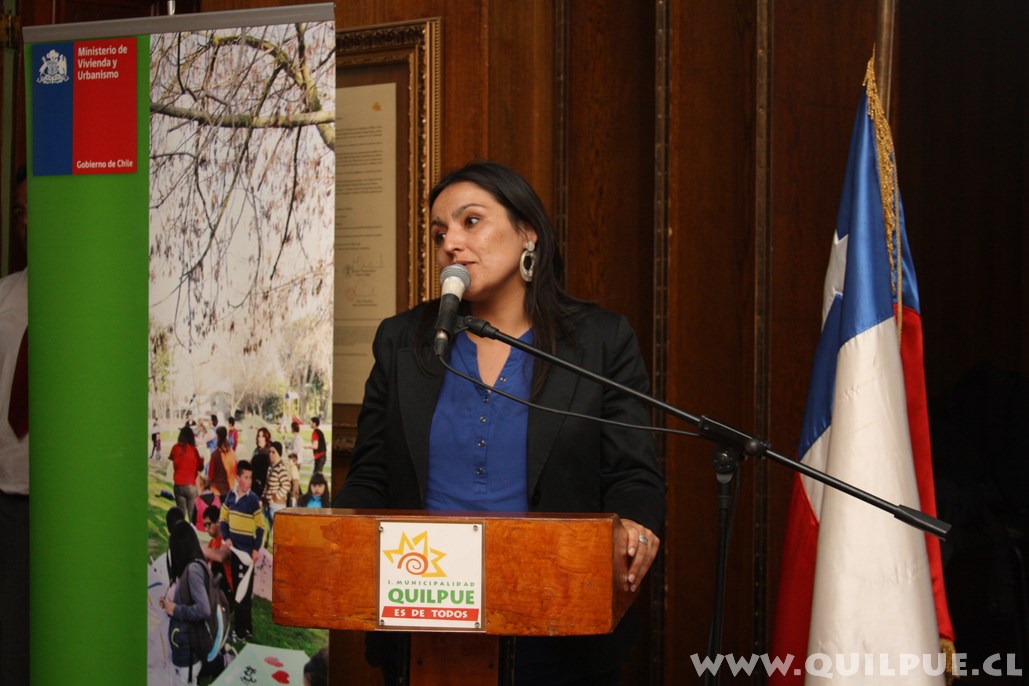A woman, approximately 40 years old, stands centered on a stage behind a wooden podium, addressing an audience with a microphone. She is dressed in a blue shirt under a black jacket, complemented by large, dangling hoop earrings, and wears a ring on her left hand, which rests on the podium. The wooden podium bears a white insignia with Spanish text. Flanking her to the right is a flag featuring the colors red, white, and blue, and a prominent star, suggesting it might be the Chilean flag. To her left, a billboard displays an image of several people outdoors, possibly students at a university, with the headline "Ministerio de Vivienda y Urbanizo" and a URL, "www.quilpue.cl," indicating a Chilean context. Behind her, the setting includes a door and a wooden-panel wall adorned with a cut-off plaque, reinforcing the indoor and possibly institutional environment of the scene.